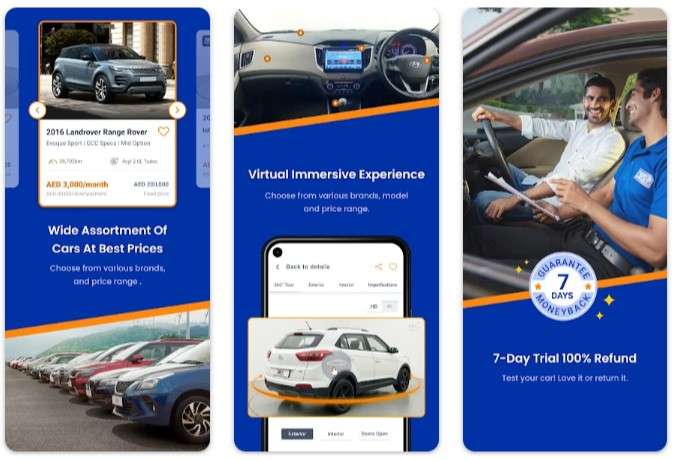This image features three distinct advertisements pertaining to automobiles, all from the same company, set against a predominantly blue World War II-themed background. 

The leftmost ad showcases a gray 2016 Land Rover with a blurry inscription underneath that reads "AED 2,000-3,000/month" in black. Above, in white text, it says, "Wide assortment of cars at best prices." The vehicles are lined up diagonally, presenting a variety of models from different brands.

The middle section highlights the interior of a car, focusing on a steering wheel positioned on the right side, indicating that the advertisement is likely not intended for an American audience. Below, in white text, it reads, "Retro immersive experience. Choose from various brands, models, and prices."

The rightmost ad displays a black phone overlaying an image of a white car. Adjacent to it is a depiction of two people inside a car; the driver, dressed in a white shirt, is positioned on the right side and is speaking to a boy in a blue shirt on the left. A circle with a bold claim offers a "7-day trial, 100% refund," and a message in white declares, "Test your car. Love it or return it."